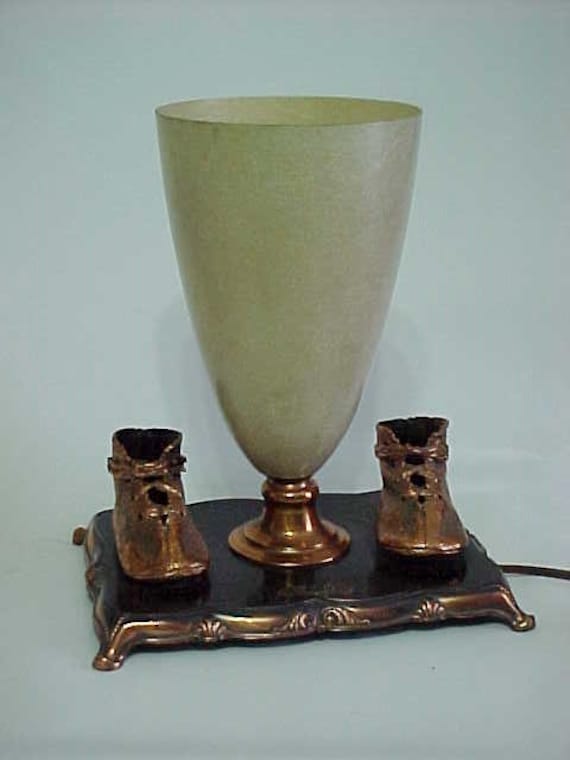The image depicts an antique brass lamp with a unique and intricate design. The lamp stands on an ornate rectangular base, featuring decorative flowery and shell-like embellishments and small feet that give it stability. At the center of the base is a circular brass pillar extending upwards into a light green cup-shaped lampshade, which is slender at the bottom and widens at the top, appearing empty. Flanking the pillar on either side are two hollow brass baby shoes with lacing, suggesting they might have been bronzed baby shoes. The top of the base is black, matching the black cord running from the lamp. The lamp casts a shadow on the light gray background, highlighting its antique patina and detailed craftsmanship.